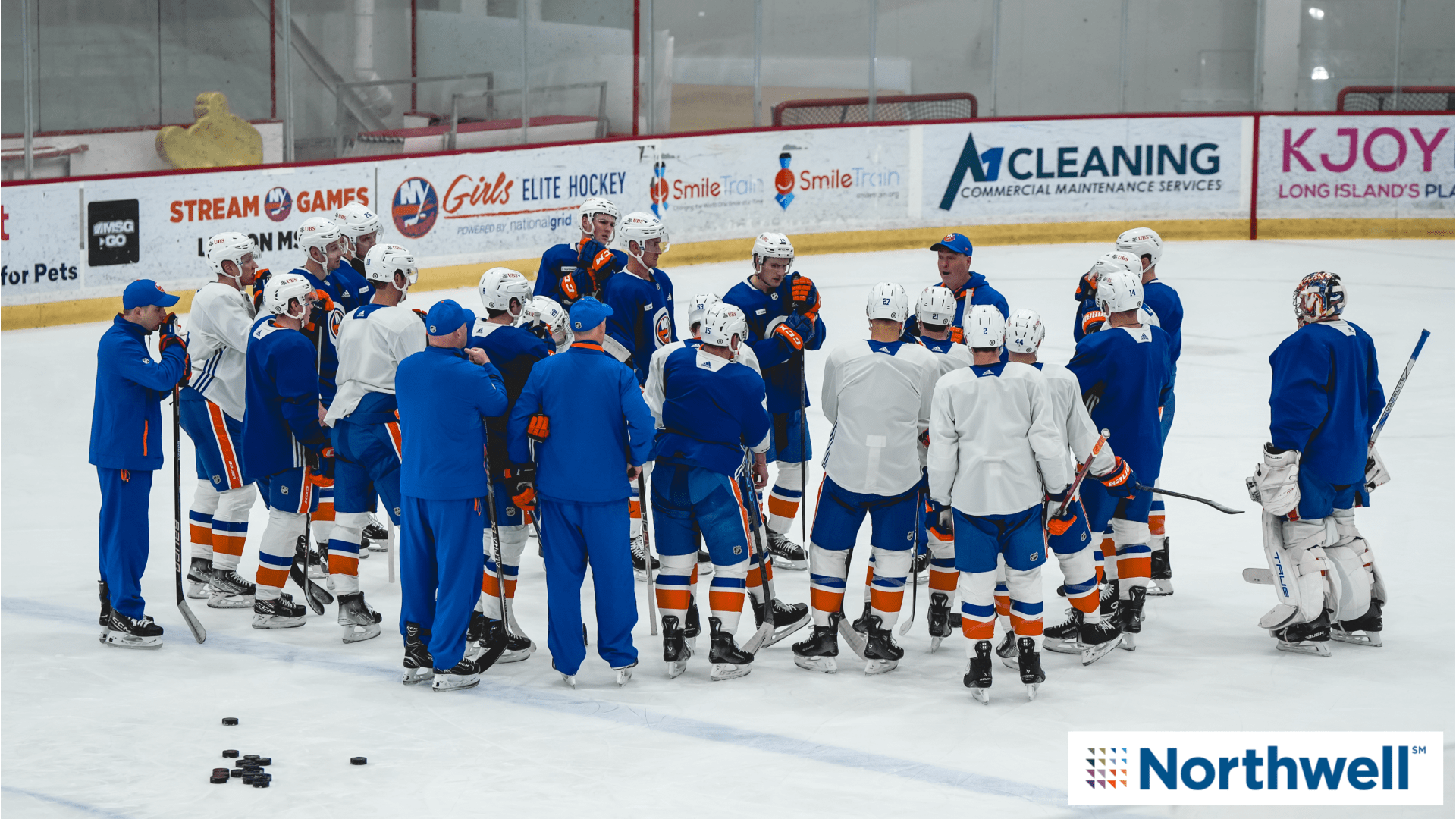The photograph depicts a hockey team having a meeting on the ice rink. The players are huddled closely together in a circle formation, engaging in discussion. They are wearing white jerseys with blue pants, accented with white and orange stripes, while the coaches are distinguished by their blue jerseys and white jackets with white pants. A pile of hockey pucks is visible on the ice in the lower left corner. In the bottom right corner, the text "Northwell" is prominently displayed. Surrounding the rink are several advertisements, such as Stream Games, New York with a hockey stick, Girls Elite Hockey, Smile, A1 Cleaning and Commercial Maintenance Services, and K-Joy Long Island. A glass wall can be seen above these advertisements, enclosing the rink area.